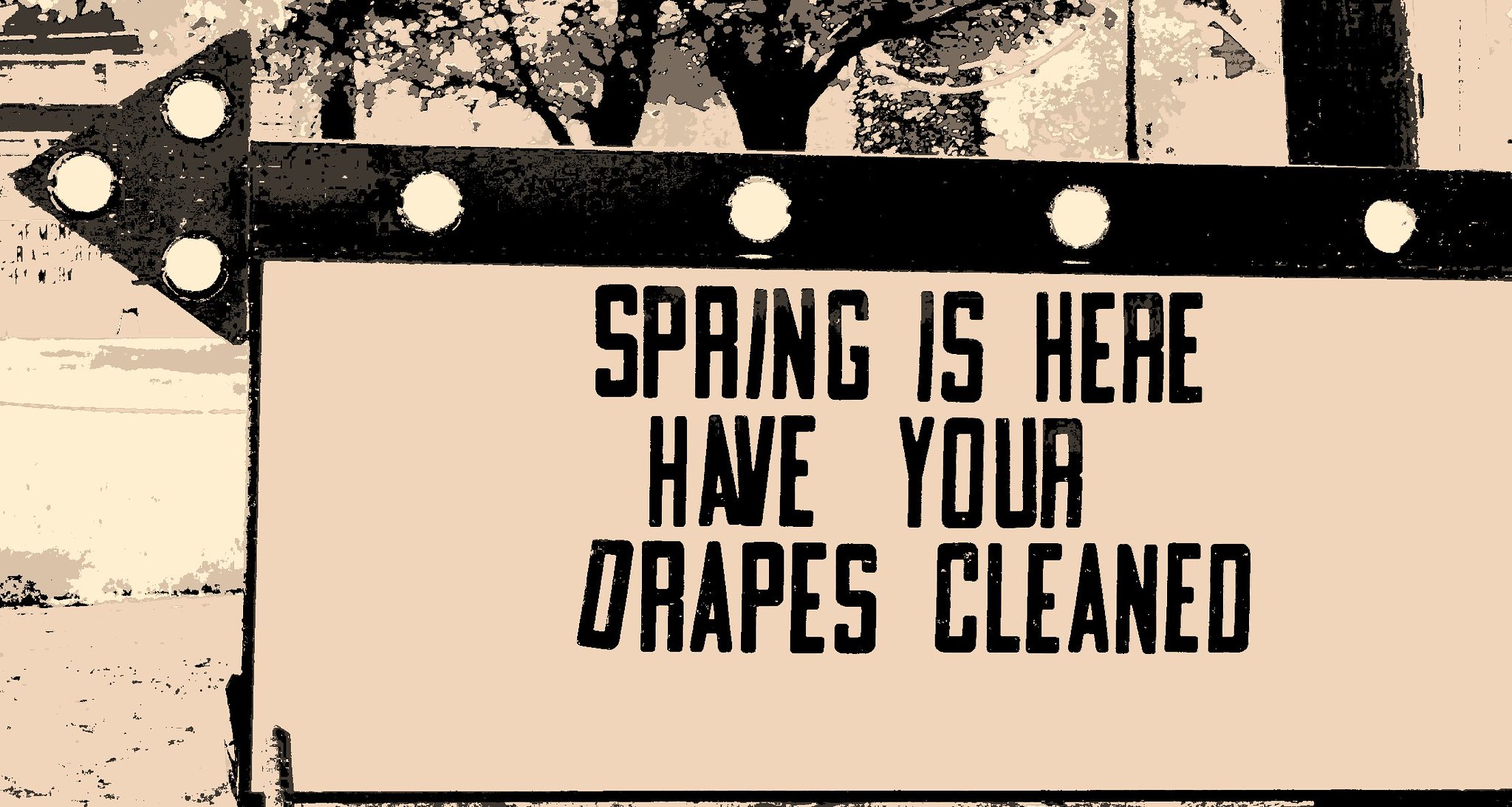This black-and-white photograph, subtly tinted in green and brown for an antique look, captures a landscape-oriented scene featuring a prominent outdoor letter board sign. The sign, positioned slightly to the right, extends three-quarters towards the left and features three lines of bold black text against a white background, stating: "Spring is here, have your drapes cleaned." Above the sign is a distinct black arrow pointing to the upper left, embellished with seven spaced-out circular lights—four on the main part and three within the triangular tip. The background showcases a high-contrast mix of trees and potentially distant buildings, partially obscured by a posterized effect that gives a distorted, digitized appearance. A portion of a tree is visible on the right side, behind the sign, adding to the textured depth of the scene. The overall image exudes a vintage, slightly surreal atmosphere, possibly indicating an advertisement outside a business such as a laundromat or upholstery cleaner.